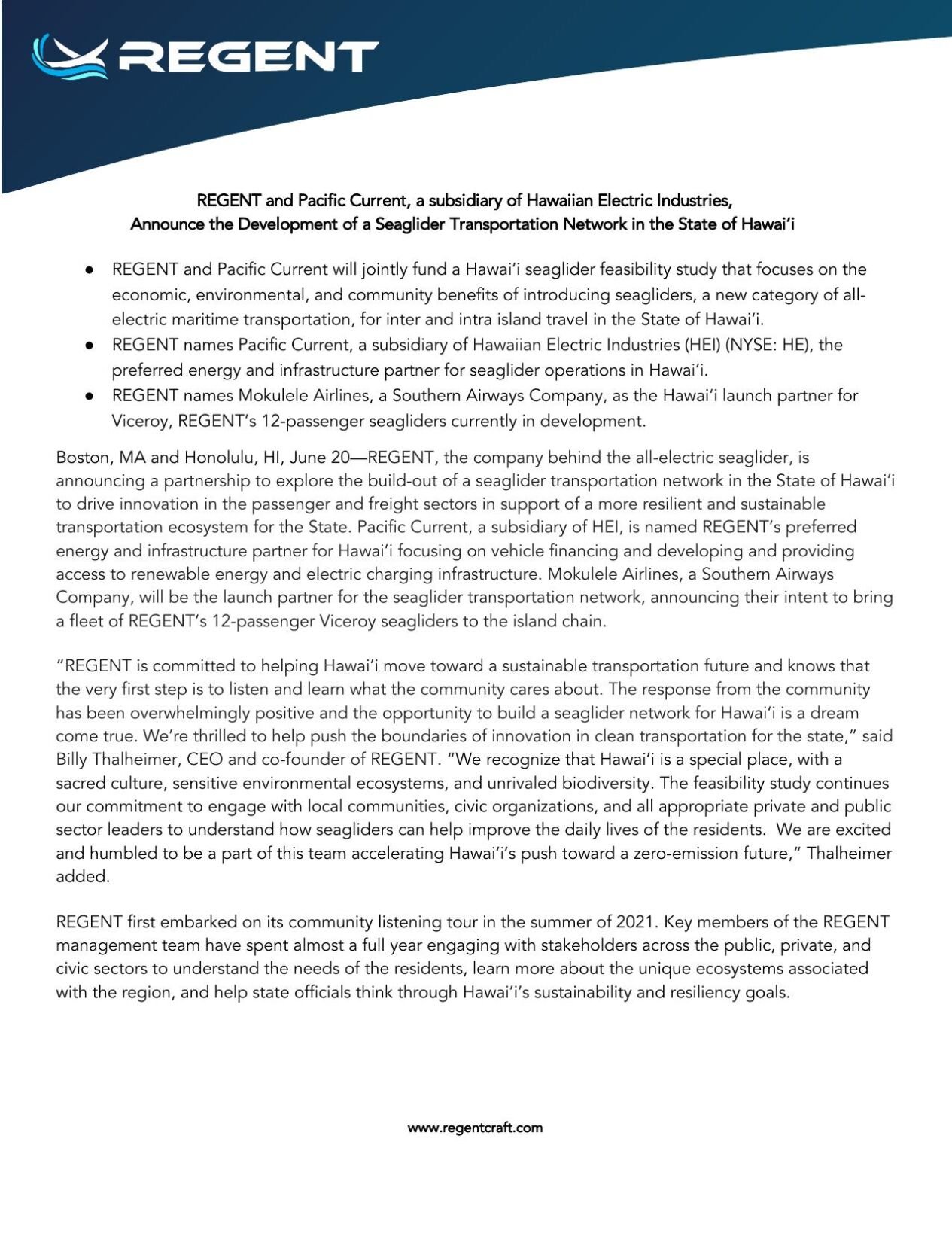An image captured from a website, titled "Regent," prominently features a blue-shaded section in the upper left corner with the word "Regent" displayed. The design resembles a sea with a bird, wings raised, possibly intended as a logo or emblem. The main announcement reads: "Regent and Pacific Current, a subsidiary of Hawaiian Electric Industries, announced the development of a sea glider transportation network in Hawaii." The description elaborates on the collaboration, revealing that Regent and Pacific Current will finance a feasibility study for the Hawaii sea glider, assessing its economic, environmental, and community benefits. The image further highlights the introduction of sea gliders, a new electric maritime transportation medium for inter- and intra-island travel in Hawaii. It designates Pacific Current as the preferred energy and infrastructure partner for sea glider operations in Hawaii and names Mokulele Airlines, a Southern Airways company, as the launch partner for Viceroy, Regent's sea glider. The detailed account is spread over three large paragraphs, concluding with the website URL www.regentcraft.com.